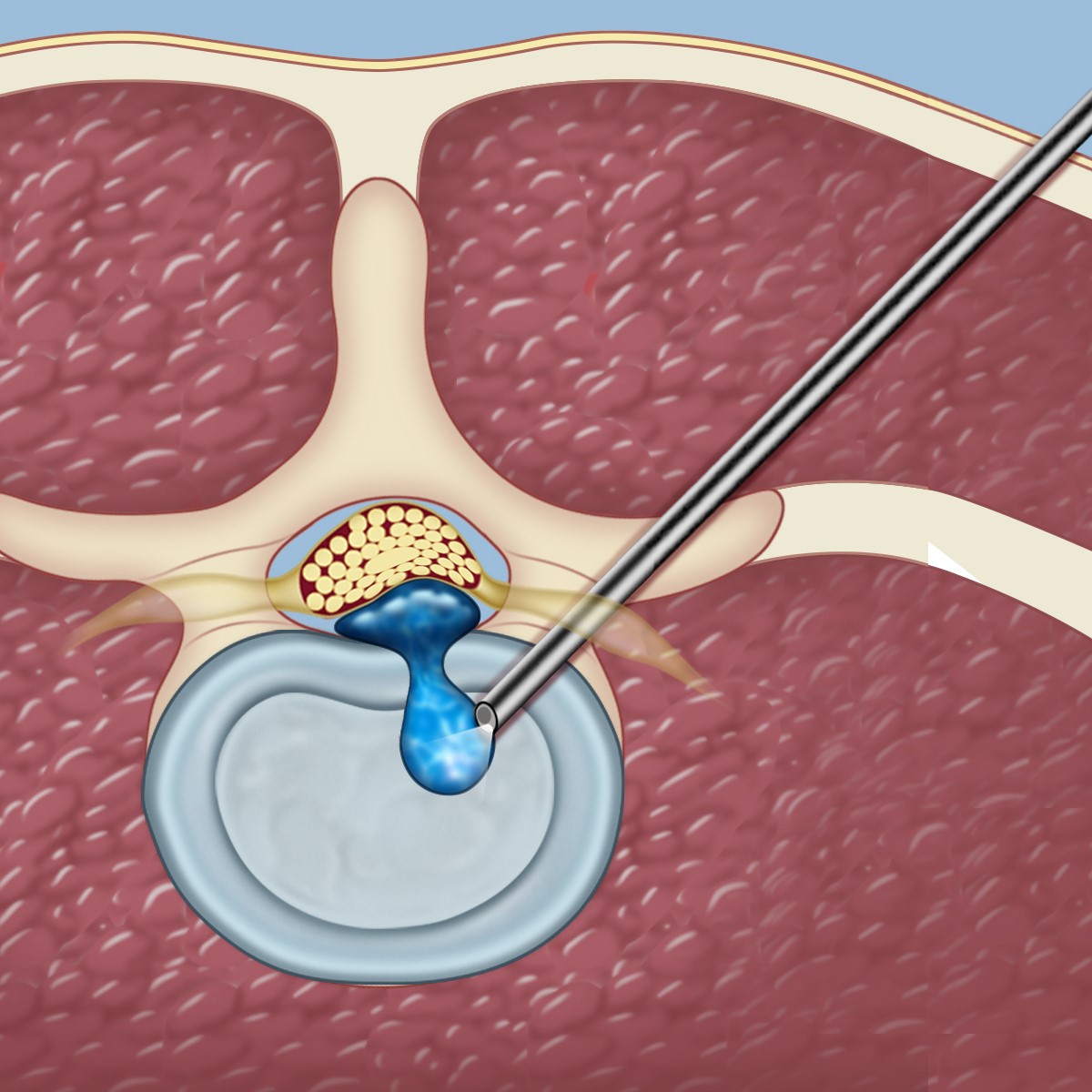The image is a stylized and realistic medical diagram, likely intended for educational purposes. It depicts a prone patient with a large, detailed needle inserted between the vertebrae, aspirating fluid from a cyst. Above the needle, a pale blue area represents air and is followed by a thin yellow layer symbolizing the skin. Beneath this layer, a light yellow color indicates fatty tissue, which overlays a representation of blood vessels and other bodily components. The needle extends deep into the body, reaching a light blue cell within a vertebra, possibly to relieve pressure on the spinal column. The image combines anatomical accuracy with a somewhat cartoony style, showing various structures in cross-section, including white and red areas representing different tissues and the path of the needle.